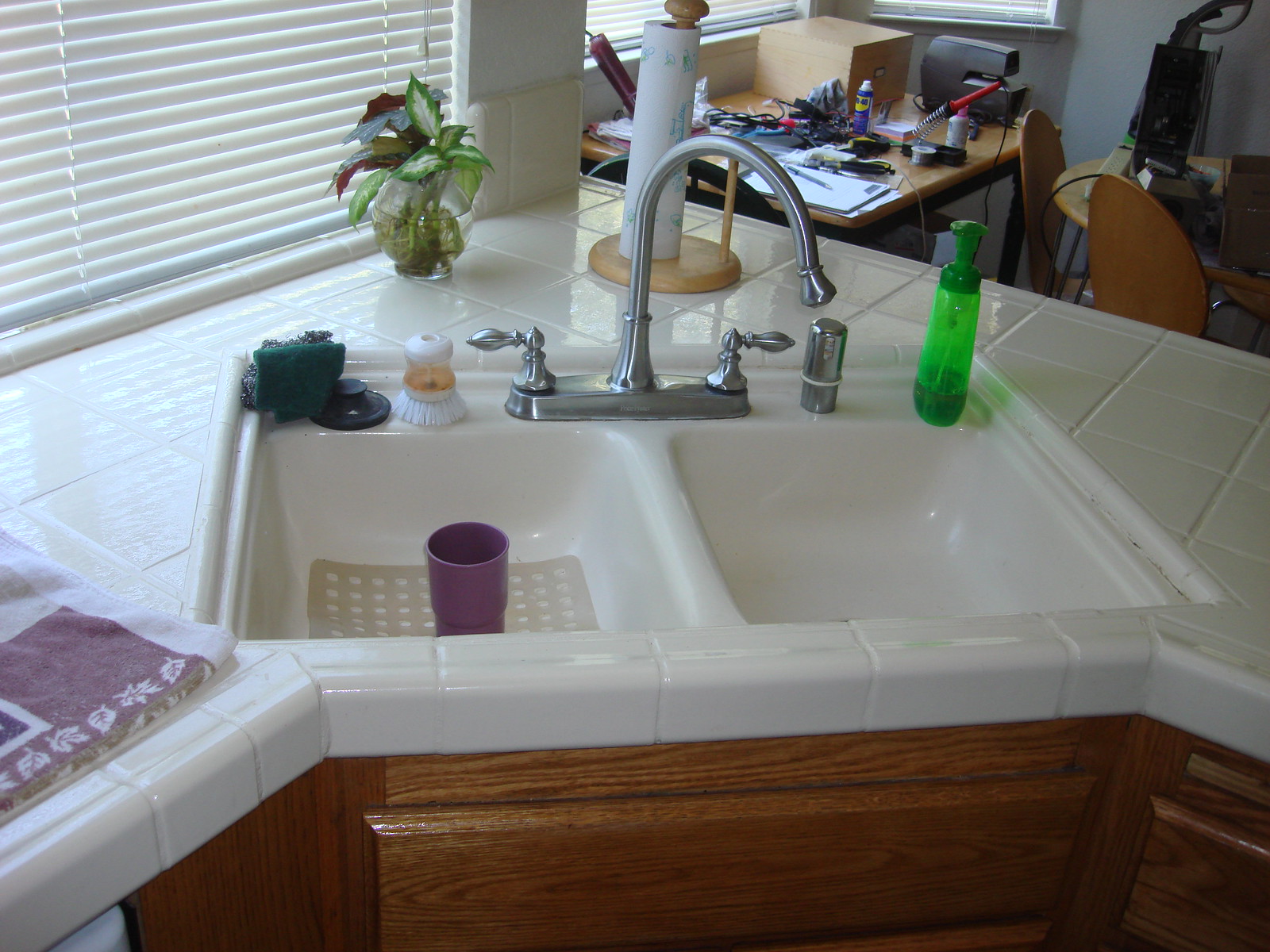The image showcases a bustling and somewhat cluttered kitchen area. Dominating the scene is a tiled countertop featuring a double kitchen sink with basins on the left and right. In front of the sink, a countertop stretches out into a workspace, crowded with various tools and materials used for working, drawing, and gluing, creating a scene of creative disarray. Adjacent to this workspace is a round table accompanied by two chairs, on which sits an apparatus that appears to be a vacuum cleaner attachment. 

On the left side of the countertop, a cloth—reminiscent of a tablecloth—lies casually. Positioned within the sink area, a handheld dish scrubber and a green bottle of soap are ready for use. Further along the counter, past the sink, there is a paper towel holder and a charming little plant that adds a touch of greenery to the otherwise industrial scene. This detailed snapshot captures a functional yet lively kitchen space, teeming with both everyday household items and creative chaos.